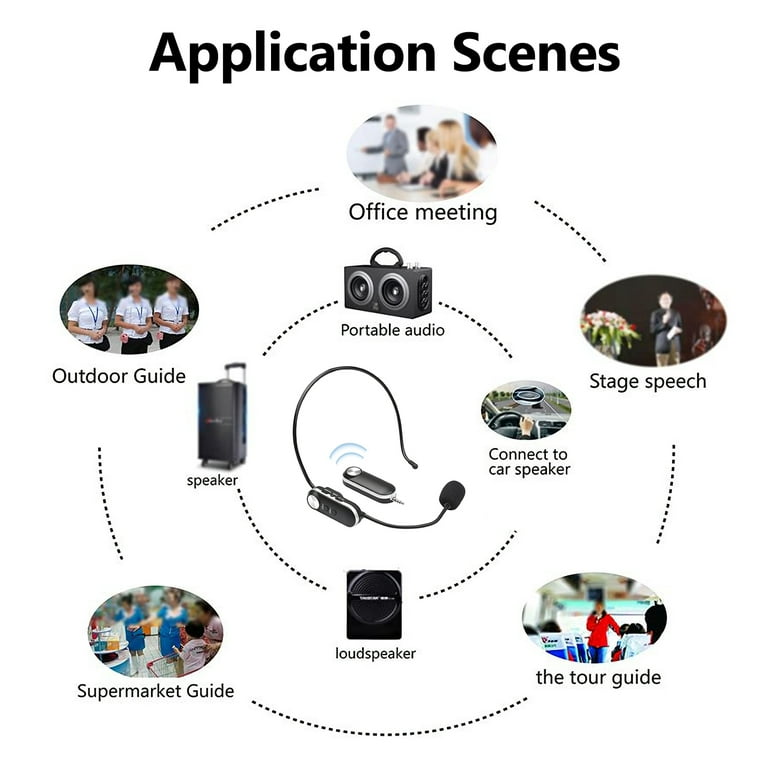The image features a detailed diagram on a solid white background with bold black letters at the top stating "application scenes." Below this heading, the diagram is arranged in a circular format, showcasing various scenarios where the product, presumably a wireless audio device such as a headset, can be utilized. At the top of the circle, an oval image labeled "office meeting" depicts people engaged in a meeting. From here, dashed lines extend to the right and left. The right side labeled "stage speech" shows a man speaking on stage with flowers in the background, while the left side labeled "outdoor guide" features individuals dressed for a summer camp environment. Further extending downwards, the diagram on the lower left depicts "supermarket guide" showing workers in a grocery store, and the lower right side shows "the tour guide" with a woman in a red jacket speaking to a group.

An inner circle within the larger one contains additional labeled graphics representing various audio applications. At the top, beneath "office meeting," is "portable audio". Extending downward with dashed connections are "speaker" to the upper left, "connect to speaker" to the right, and "loudspeaker" at the bottom. These various areas are interconnected with dashed lines, converging towards a central image of the wireless headset, symbolizing the versatility of the device in multiple environments and setups.